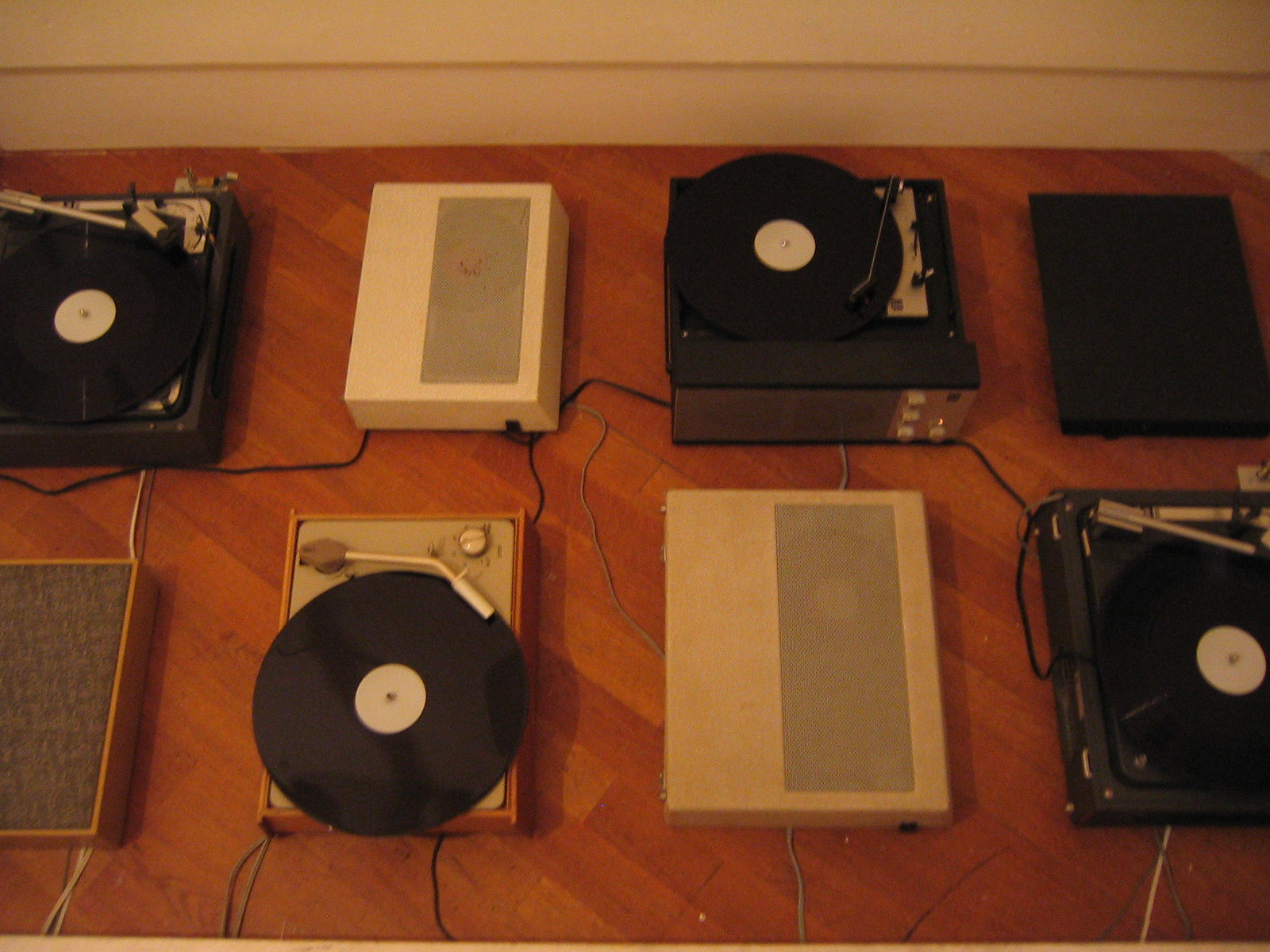The photograph captures a nostalgic scene of four vintage record players and their corresponding speakers, all arranged neatly on a diagonal hardwood floor. The floor has an amber hue, suggesting it may be an older image or one with a retro filter. The upper part of the photograph shows a white-painted wall with a trim matching the floor’s hue.

Starting from the bottom left, the first record player has an orange wood finish with a beige interior, paired with an orange speaker featuring a gray cover. The next set includes a white record player with a gray plastic speaker cover, sitting beside a tan speaker with a gray cover. The rightmost pair includes a black record player with a black stem, accompanied by a black speaker. Intricately placed vinyl records—ranging from dark brown to black—rest on each turntable. The overall arrangement of the components is such that they alternate: record player, then speaker, followed again by record player and speaker in a contrasting but harmonious vintage aesthetic.